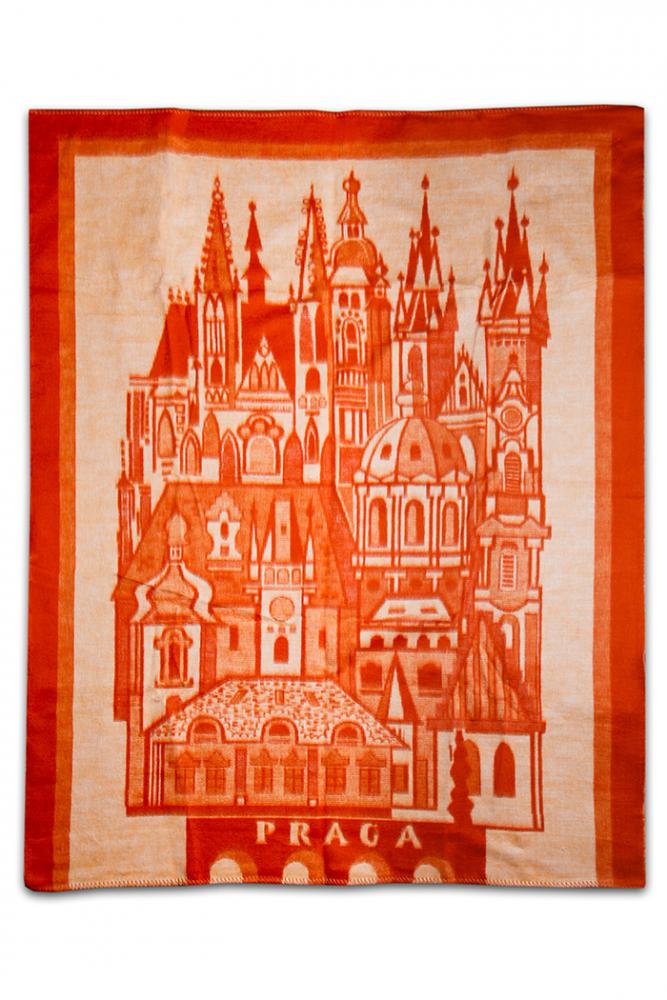The image is of a detailed tapestry with an off-white, almost tan background, encased in a dark red border, and further framed by an inner orange line. Dominating the tapestry is an intricate depiction of various buildings, densely packed together, showcasing a diversity of architectural styles. Some rooftops are dome-shaped, others are triangular or spiky, and many exhibit ornate features like stone mosaics. Centrally, there's a prominent red structure with semi-circular cutouts, bearing the inscription "Praga" at the bottom, indicating a reference to Prague. The buildings, unified under a consistent color palette of red, orange, and tan, create a cluttered yet grand visual. The tapestry, designed with reddish ink, gives an impression of a cohesive yet diverse cityscape, blending castle-like structures with multiple levels, towering spires, and numerous windows and doors, enhancing its majestic and powerful appearance.